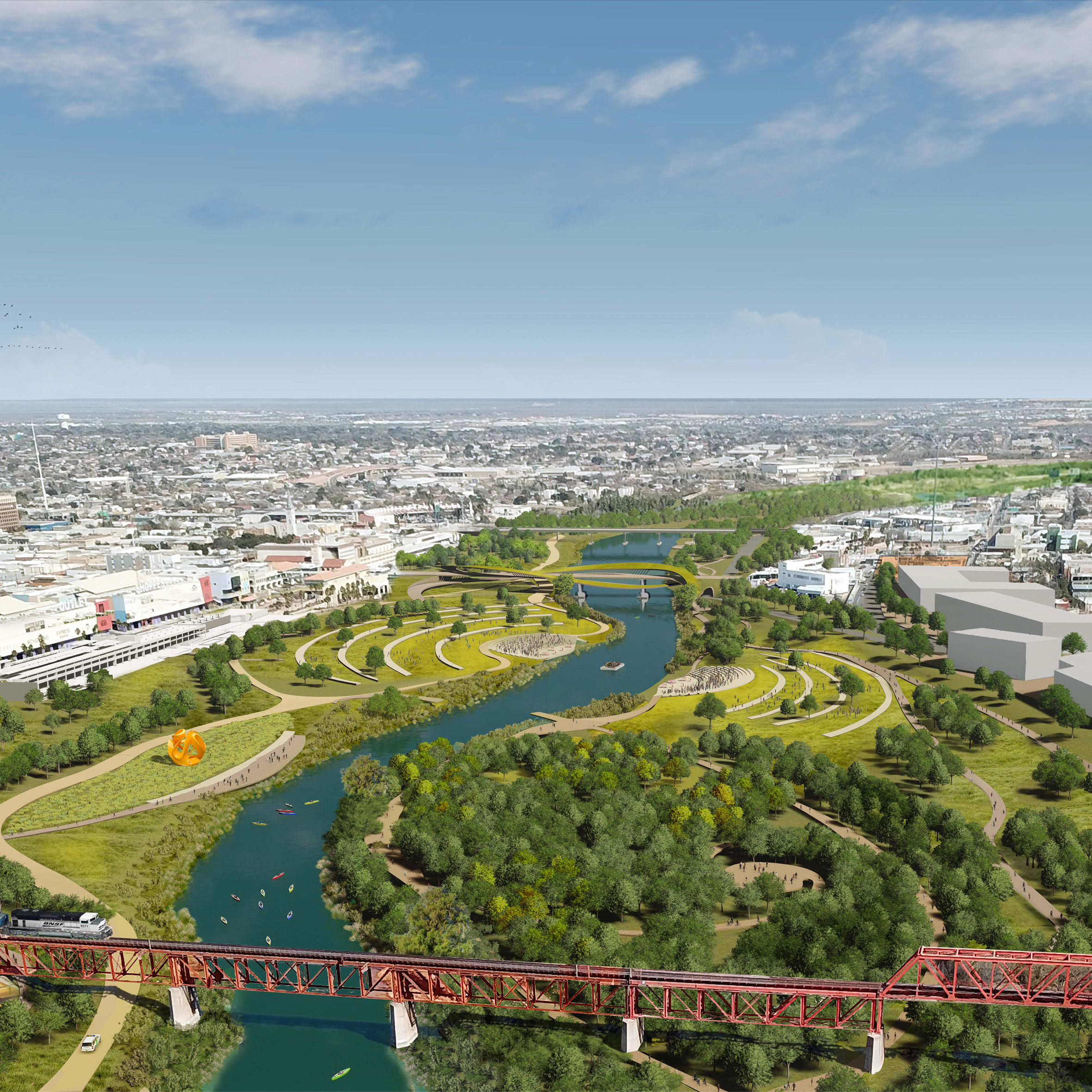This detailed aerial photo depicts a vibrant cityscape bisected by a winding blue-green river. Dominating the foreground is an iconic two-story red bridge designed for trains, with a white train visibly crossing it. The water below bustles with activity, including people kayaking, adding to the dynamic atmosphere. On the right side of the river, lush greenery and trees are visible, providing a picturesque contrast to the more urban setting on the left side where paths and roads can be seen. Adding a splash of color, an orange spherical art sculpture sits near the river, drawing the eye. The buildings in the background are primarily white, suggesting it might be a significant or capital city. The cityscape extends to the horizon, where train yards and various buildings stand against a backdrop of blue skies and scattered clouds. The image captures a lively, populous area with numerous sidewalks and pathways, indicating it's a popular spot for both locals and visitors to enjoy outdoor activities and the scenic river views.